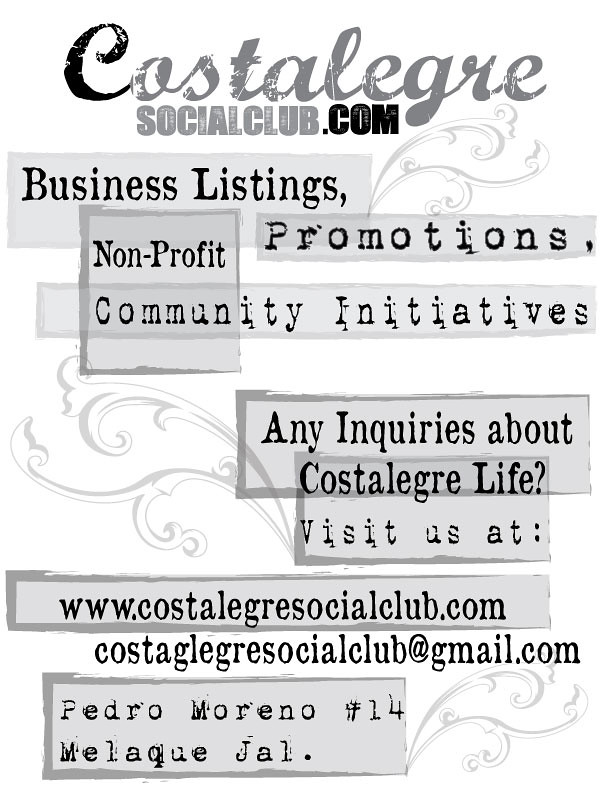The image is a tall rectangular digital advertisement with a completely white background adorned with light gray, swirly floral designs. At the top, it prominently features the website "Coastallegraysocialclub.com" in intentionally damaged-looking gray font. The text is repeated below in a combination of bold, all capital sans serif fonts and graceful gray cursive, with "SocialClub.com" highlighted in gray and ".com" in black.

Beneath the main headline are several light gray rectangles with handwritten-style gray borders, each containing phrases: "Business Listings," "Promotions," "Non-Profit," and "Community Initiatives." The advertisement prompts any inquiries about "Costa Alegre life" and directs visitors to "www.coastallegraysocialclub.com" or to email "Costalegraysocialclub@gmail.com." The contact information concludes with a reference to Pedro Moreno, at number 14, in Malak JAL.